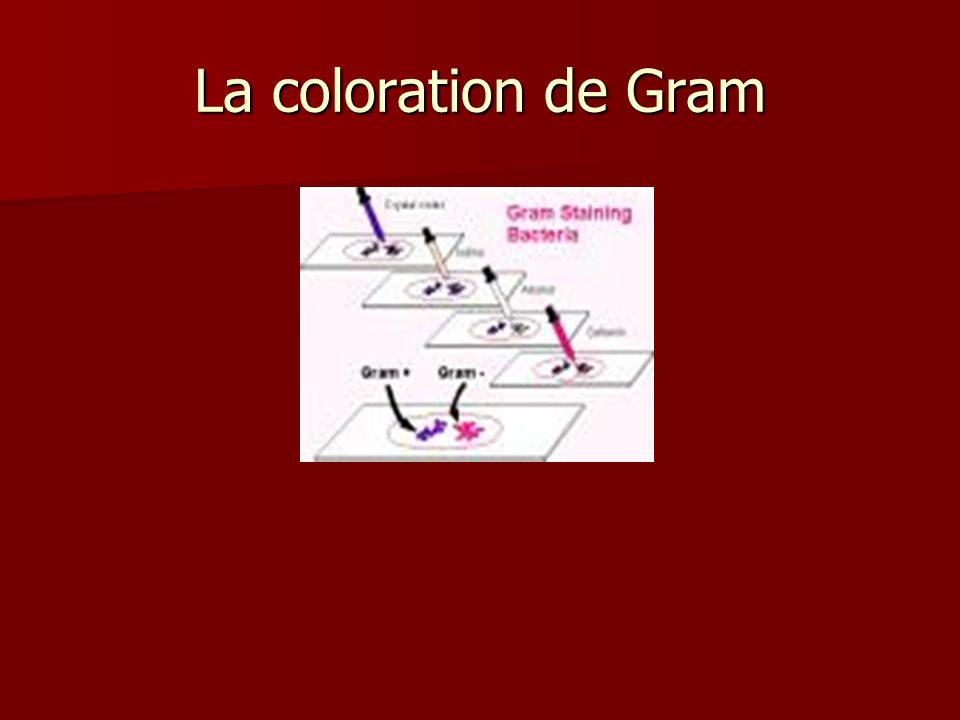The image resembles a slightly wider-than-tall poster or infographic with a maroon or dark red background. At the top, there is a text in yellow or beige that says "La Coloration de Gram" in French. Below this title, there's a white box containing an illustration. This illustration appears to depict four syringes or eyedroppers above a Petri dish or microscopic slides, seemingly involved in the process of Gram staining bacteria. The text within this box also reads "Gram Staining Bacteria." The syringes are shown dispensing various colored liquids ranging from white to purple and pink, emphasizing the bacterial staining process. Overall, this appears to be a scientific educational graphic explaining the Gram staining technique in bacteriology.